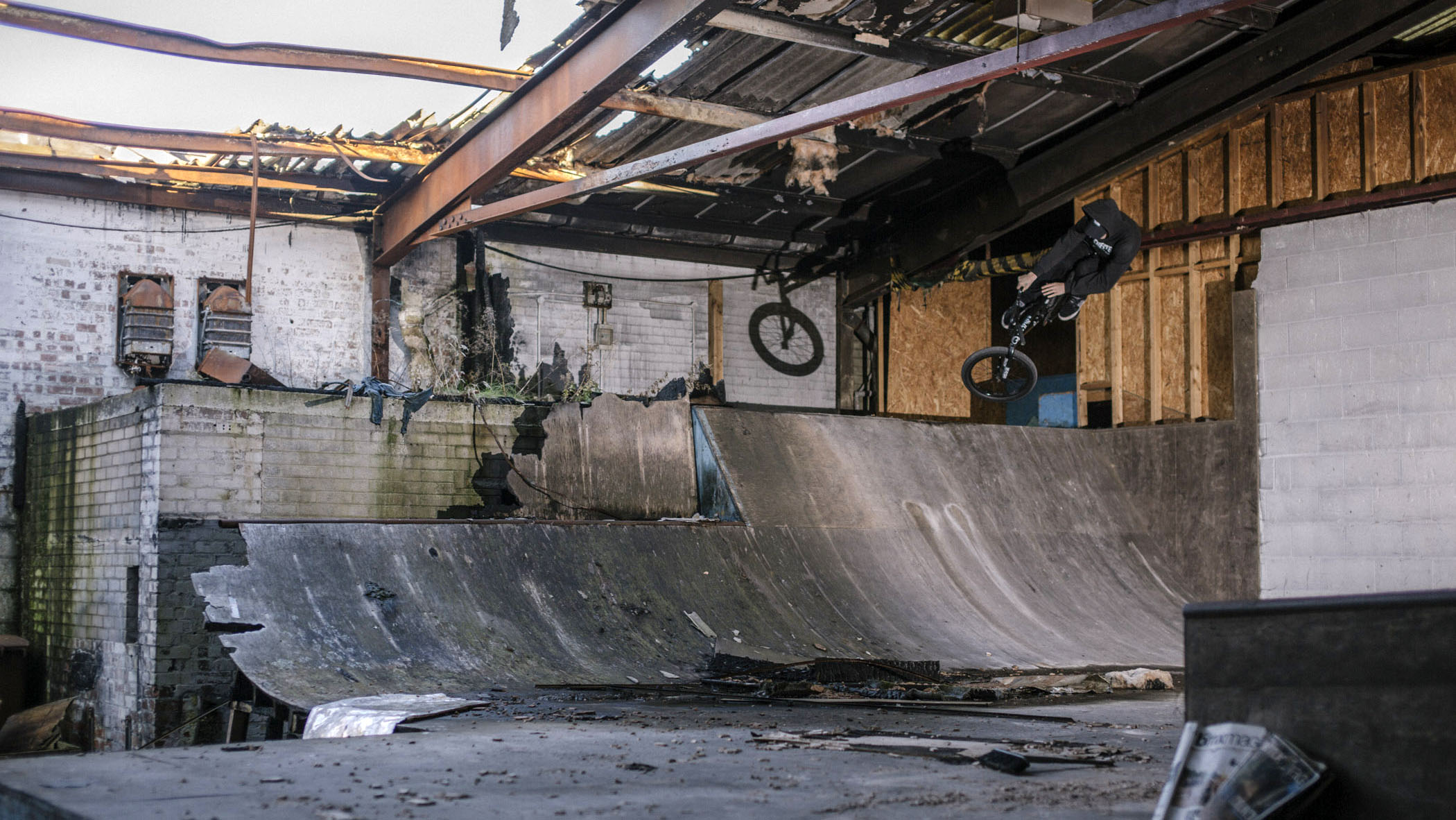In this photo, taken outside during the day, we see the ruins of an old structure that some imaginative bikers have repurposed into a makeshift BMX playground. The building, with its open roof lines and exposed metal joists, frames the sky beyond, giving a stark reminder of its dilapidated state. Most of the roof is missing or caved in, with remnants of metal roofing precariously hanging or littering the ground.

At the center of the scene, two BMX bikers are captured in midair, parallel to each other, performing tricks. The biker on the right is dressed in all black, complete with a black baseball cap, and his bare hands grip the handlebars tightly as his wheels are turned to the left. Just beside him, another bike mirrors the motion, although the rider is less visible. The ramp they are using is a makeshift setup built over a decaying warehouse structure with a large garage door. The grey ramp is falling apart, with chunks missing and debris scattered around.

In the background, to the left of the ramps, stands a brick building adorned with what looks like old air conditioning units, further accentuating the rundown atmosphere. This repurposed playground, with its retro, 90s-esque photograph coloring, offers a gritty yet resourceful glimpse into the creativity of these young bikers making the best of their urban surroundings.